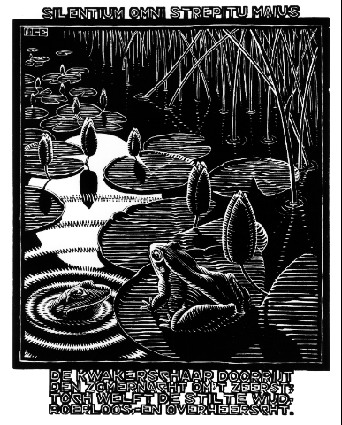The image is a meticulously detailed black-and-white ink drawing of a tranquil pond scene. The artwork is titled with text at the top that reads, "Silent Tongue Omni Strep to Madness," although the meaning remains unclear. The bottom of the image contains more squished, nearly illegible text, possibly reading, "the cow with shabba door it."

At the center of this serene pond, a realistic frog is perched on a lily pad, surrounded by numerous lily pads adorned with flower bulbs. To the left of the main frog, another smaller frog's head emerges from the water, creating three ripples that expand outward, intersecting with the main frog's lily pad and reaching the surrounding pads. The water is depicted in a deep, reflective black, with a prominent white moon casting its glow and reflections across the scene. Reeds protrude out of the pond, adding natural detail to the composition.